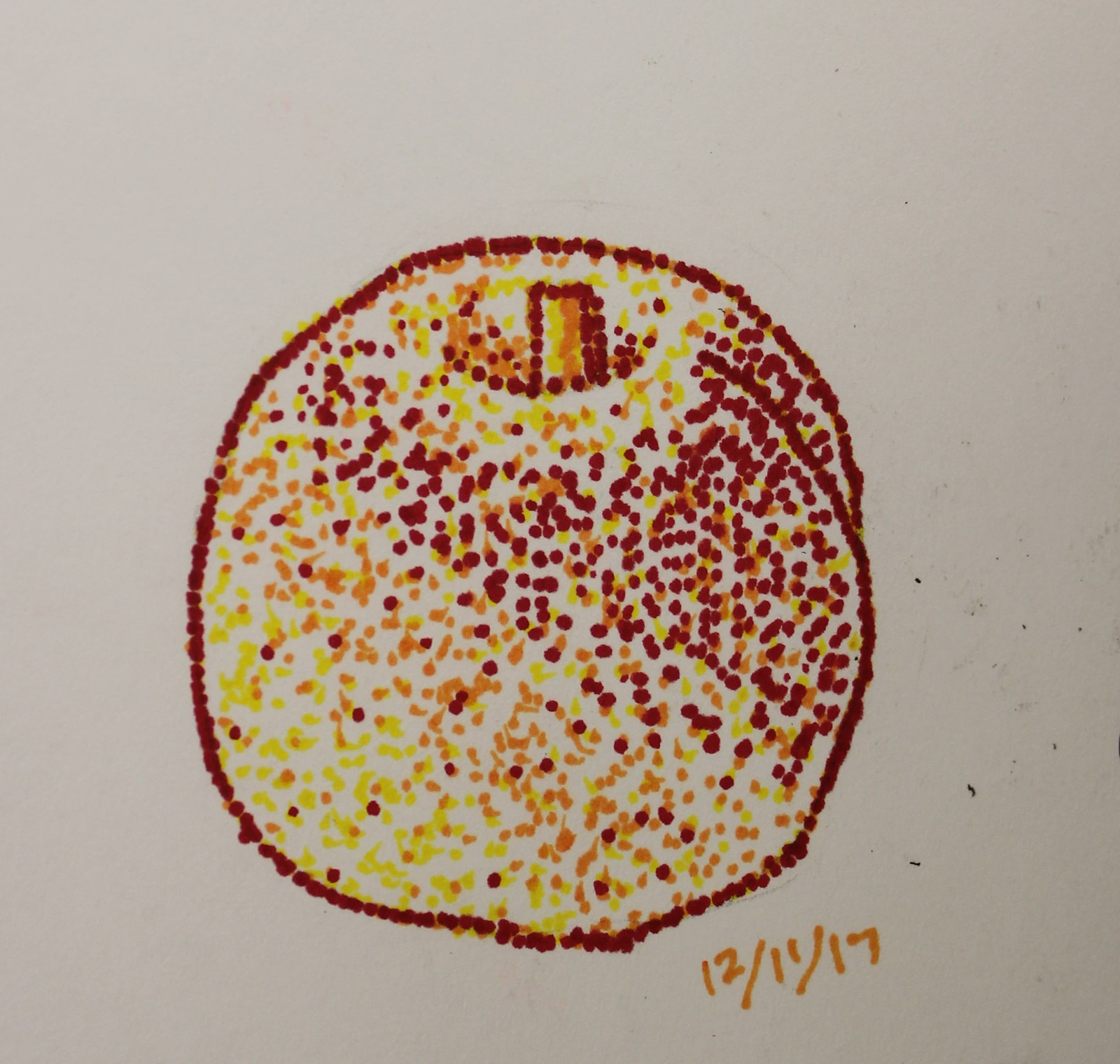This is a detailed pointillist drawing of a round fruit, possibly a peach or an apple, set against a grayish-violet background. The image is constructed entirely from dots, with a red dot outline defining its shape and adding depth and dimension. Inside the fruit, clusters of yellow, orange, and red dots create a textured, yet partially unfilled interior, leaving some areas white or blank. At the top, a short stem is also depicted using red dots. The background appears to have some smudges, adding a slight texture. An important detail is the date "12/11/17" written in orange marker on the bottom right corner of the piece.